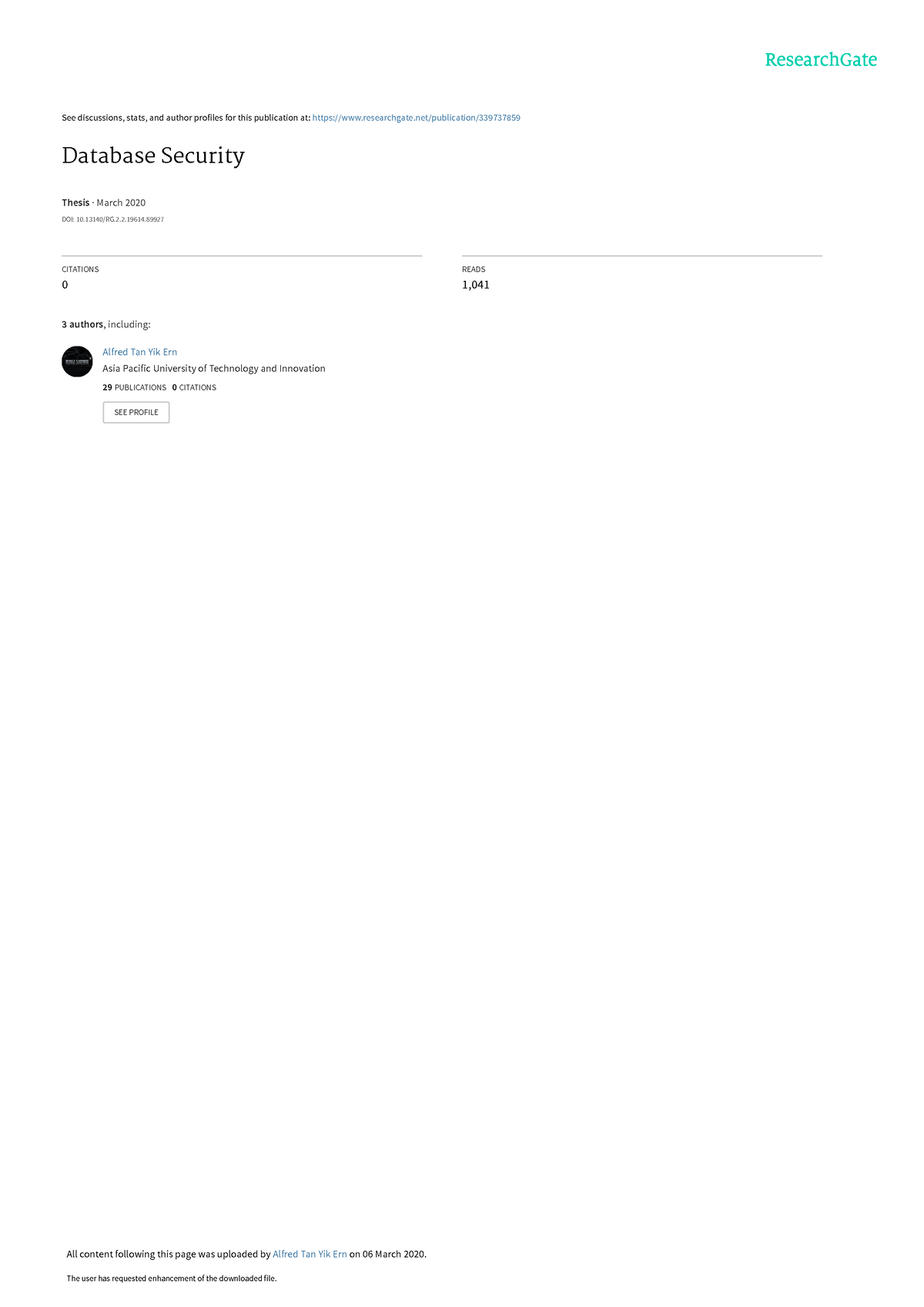Here is a refined and detailed caption for the image described:

---

The image is a screenshot from a webpage on ResearchGate, focusing on a publication related to database security. At the top right corner of the image, the ResearchGate logo is featured in teal. The main section prominently displays the title "Database Security" and underneath it, the word "THESIS" is followed by "March 2020".

Below this information are several statistics: "Citations" marked as zero, and "Reads" showing 1,041. The author details reveal three contributors, with one named Alfred Tan Yik Ern affiliated with Asia Pacific University of Technology and Innovation, listing 29 publications. The bottom of the image features a link inviting viewers to "see people," potentially leading to more information about the authors.

The URL "https://www.researchgate.net/publication/[long number]" is partially visible, indicating a direct link to the publication where further details, discussions, statistics, and author profiles can be accessed.

---

This caption maintains the informative nature of the original description while structuring it in a more concise and readable format.